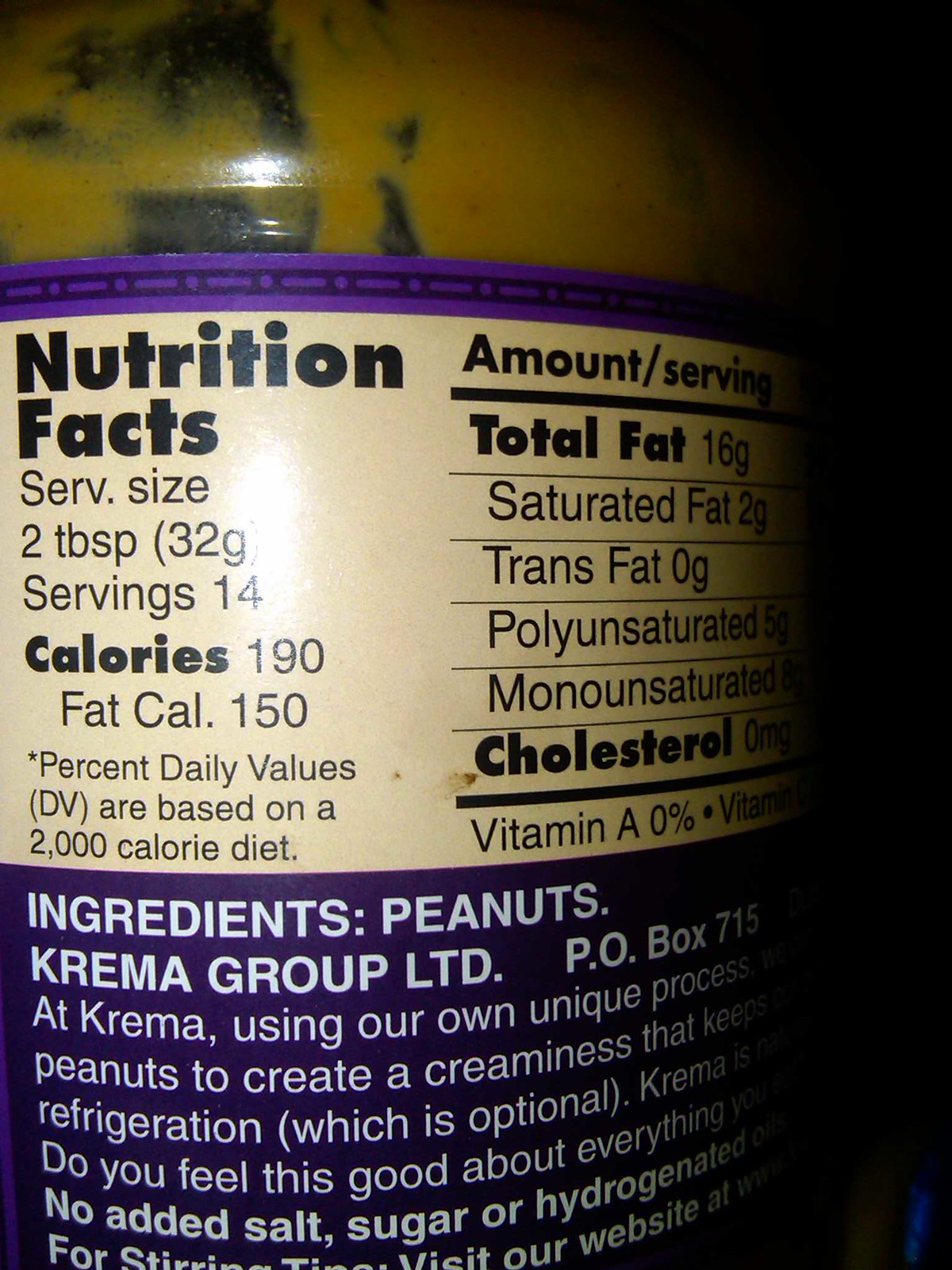In this photograph, we see the backside of a clear jar of peanut butter, showcasing its detailed nutrition label. The jar features a purple and white label, although only the rear section with the nutrition information is visible to us. Above the label, there is a noticeable residue of peanut butter on the jar. The nutrition facts panel outlines the serving sizes and detailed nutritional content of the peanut butter. Below this panel, the list of ingredients is presented, which indicates that the peanut butter consists solely of peanuts, with no additional ingredients. Further down, there is a message from the manufacturer, Crema Group Limited, stating that they are the producers of this all-natural peanut butter.